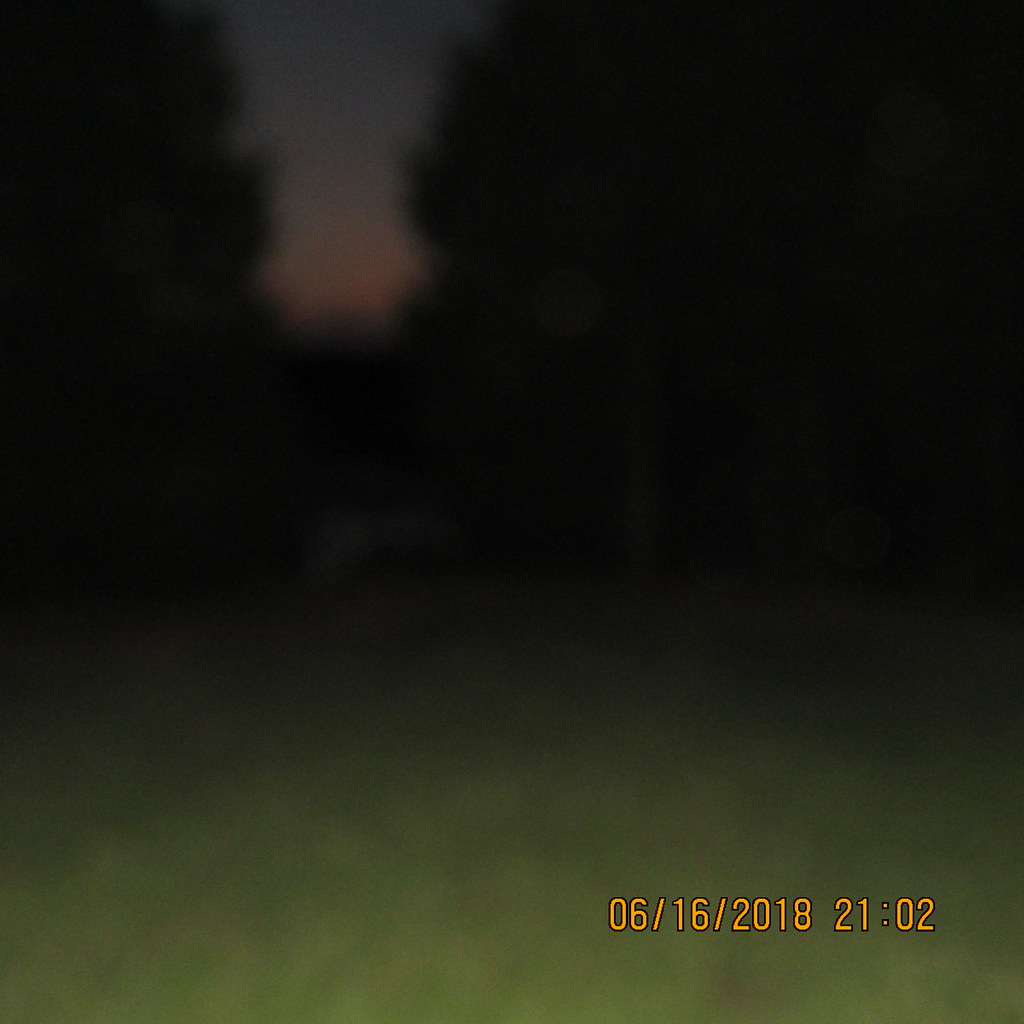This image depicts an outdoor scene captured during either the twilight period of a sunrise or the closing moments of a sunset. The sky transitions from a muted blue at the top to soft pink hues along the horizon, suggesting the softer light of dawn or dusk. In the foreground, there is a green area likely covered with grass. The background is dominated by very dark silhouettes that appear to be trees, creating a natural frame around a central gap where the sky is visible. Amidst the backdrop, there's an indistinct shape that hints at the presence of an animal, though it's challenging to identify clearly. Notably, the bottom right corner of the image features orange text displaying the date "June 16, 2018" and the time "21:02."